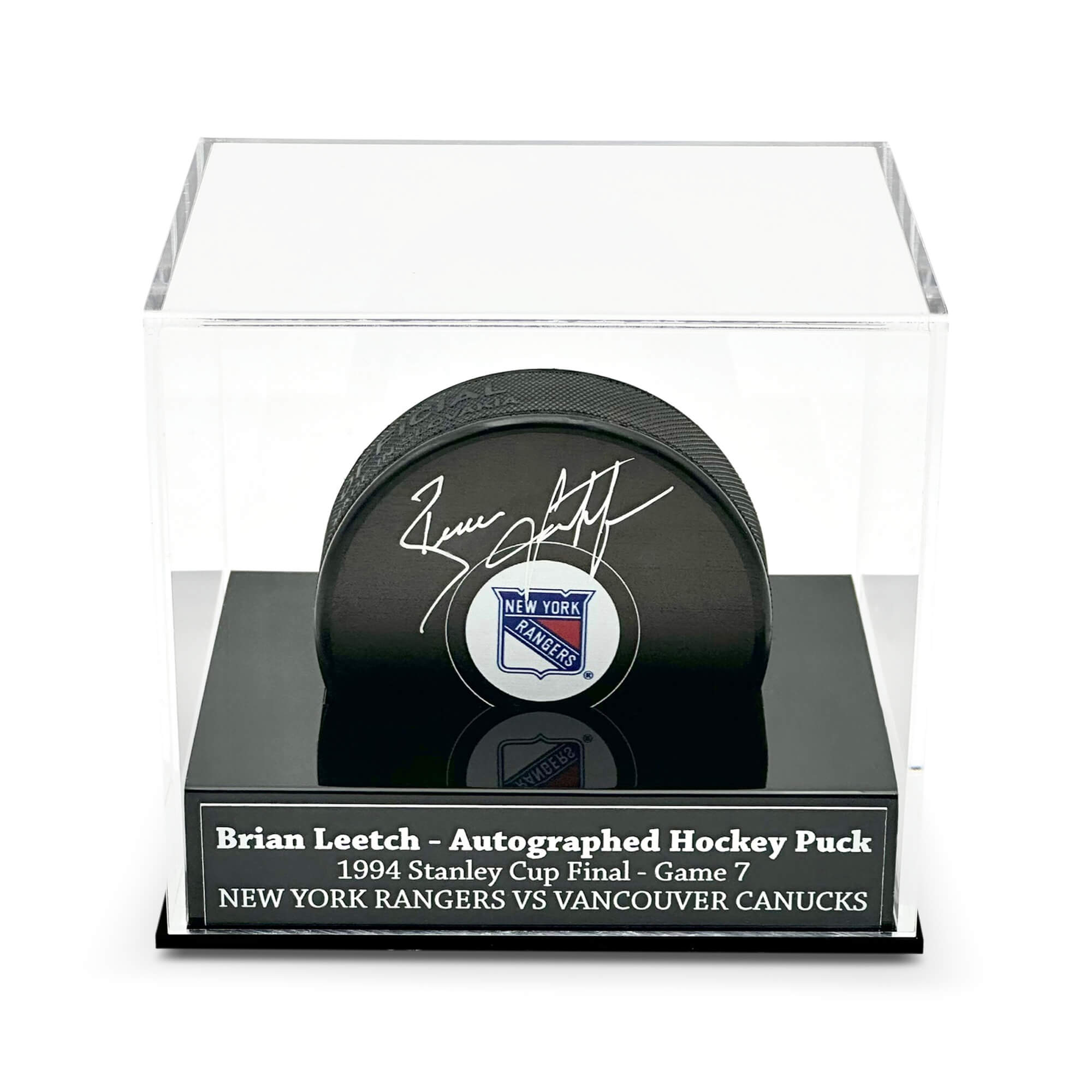The image depicts a black hockey puck encased in a clear, cubed glass display case with a black base approximately an inch and a half high. The case sits against a solid white background, accentuating the puck inside. The front of the base features a plate with white engravings that read, "Brian Leach autographed hockey puck, 1994 Stanley Cup Final, Game 7, New York Rangers vs. Vancouver Canucks." The hockey puck, which appears to be real, bears a smooth front and gripped edges, and is prominently centered in the display. It has the New York Rangers logo in red, white, and blue, and is autographed by Brian Leach in white ink. The text "Official" and other minor inscriptions are also present on the puck, though partially obscured in the image.